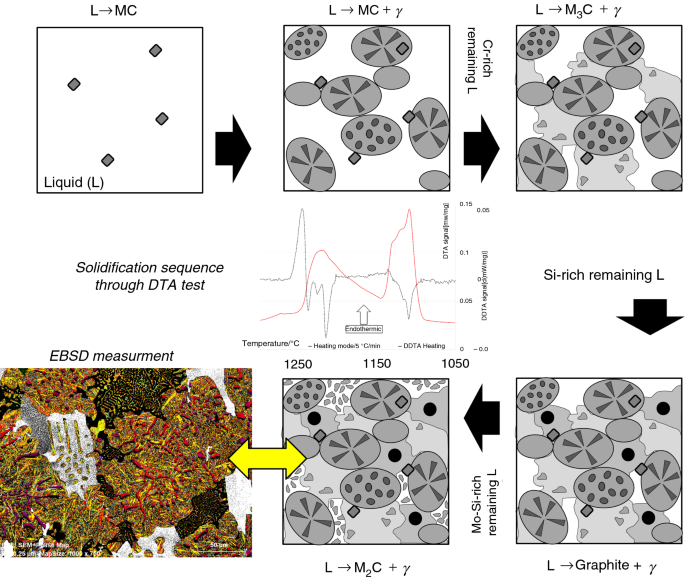The image is a square, multicolored scientific flowchart with a white background, divided into nine sections, showcasing the solidification sequence through DTA (Differential Thermal Analysis) tests. The top row consists of three black outlined squares. The leftmost square is labeled "Liquid (L)" and contains four gray diamond-shaped dots. The middle square has eight circles resembling gray and black sand dollars and chocolate chip cookies, while the rightmost square features similar circles with additional light gray shapes.

In the center of the flowchart, there is a bar graph with small, unreadable black lettering, possibly showing temperature in Celsius, and annotated with "solidification sequence through DTA test" on the left and "Si-rich remaining L" on the right. Above these annotations are complex equations.

The bottom row comprises three squares. The leftmost square is colorful, displaying an EBSD (Electron Backscatter Diffraction) measurement in shades of green, brown, tan, red, and yellow. The middle and right squares are similar to the upper right square, depicting circles, gray lighter blobs, solid black dots, and additional smaller gray kernels. The middle square, which has a yellow double-headed arrow on the left margin, mirrors the pattern above with flecked gray kernels.

Together, these elements visually describe a chemical process evolving from a liquid state to a graphite structure, ultimately represented by an EBSD measurement. Despite the complexity and scientific nature of the image, the intricate depiction and color variations provide a detailed view of the solidification sequence.